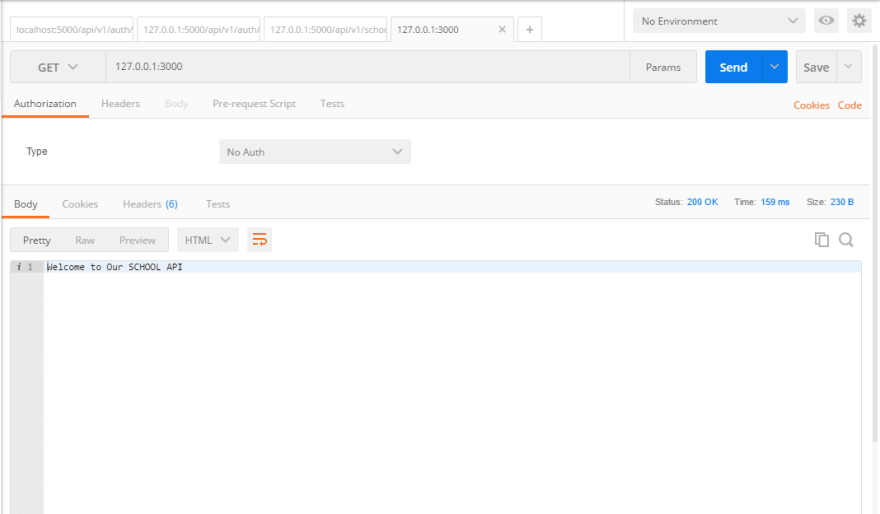The image depicts a computer screen showing search results. Multiple tabs are visible, with the active tab highlighted in a light gray background, displaying the repeated number "127.0.0.1:3000" towards the left side.

The interface shows several key elements. At the top, the word "GET" is prominently displayed, suggesting an HTTP GET request. Below this, the word "Authorization" stands out, highlighted and underlined in orange, indicating its selection. Adjacent to this are form items labeled "Headers," "Body," "Pre-request Script," and "Tests," with "Authorization" selected.

Further down, "Type" appears with a clickable block labeled "No Auth." Underneath, "Body" is highlighted and underlined in orange, followed by form items "Cookies," "Headers" (with "6" in blue parentheses), and "Tests." Below these, options labeled "Pretty," "Raw," and "Preview" are displayed in a small rectangle, with "Pretty" selected. The bottom of the screen features a blue-highlighted area with the text "Welcome to our school API."